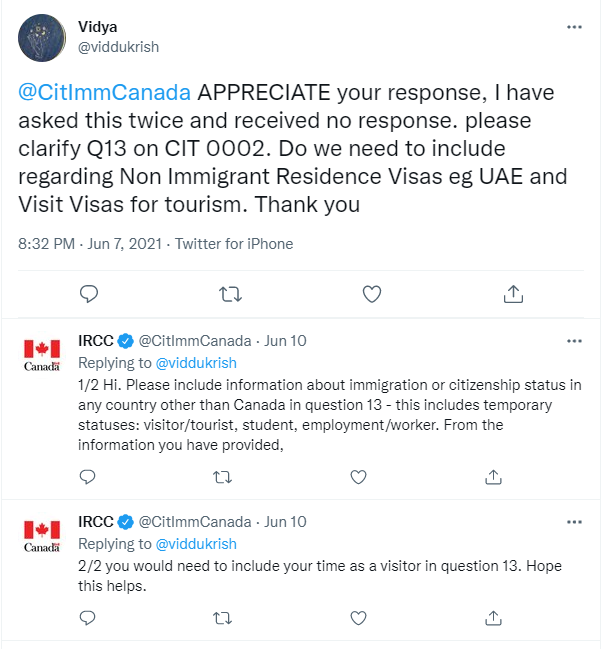**Detailed Caption:**

At the very top left corner of the image, there is a Twitter post from Vidya (@Vidyukrish). The profile icon features a blue background with a Dreamcatcher-like design in the center. On the right side of the username is the three-dot menu icon.

The original tweet reads:
 
"@sitlmncanada, APPRECIATE your response, I have asked this twice and received no response. Please clarify Q13 on CIT0002. Do we need to include non-immigrant resident visas, e.g., UAE visit visas for tourism? Thank you. 8:32 PM · Jun 7, 2021 · Twitter for iPhone."

Beneath this post, you see the comment, retweet, like, and share icons.

Below the original tweet, there is a reply from a verified account IRCC (@sitlmncanada), featuring the Canadian flag icon. The reply is timestamped June 10 and says:

"Hi, please include information about immigration or citizen status in any country other than Canada in question 13—this includes temporary statuses: visitor/tourist, student, employment/worker. Based on the information you have provided, please include your time as a visitor in question 13. Hope this helps."

This reply also has the comment, retweet, like, and share icons beneath it.